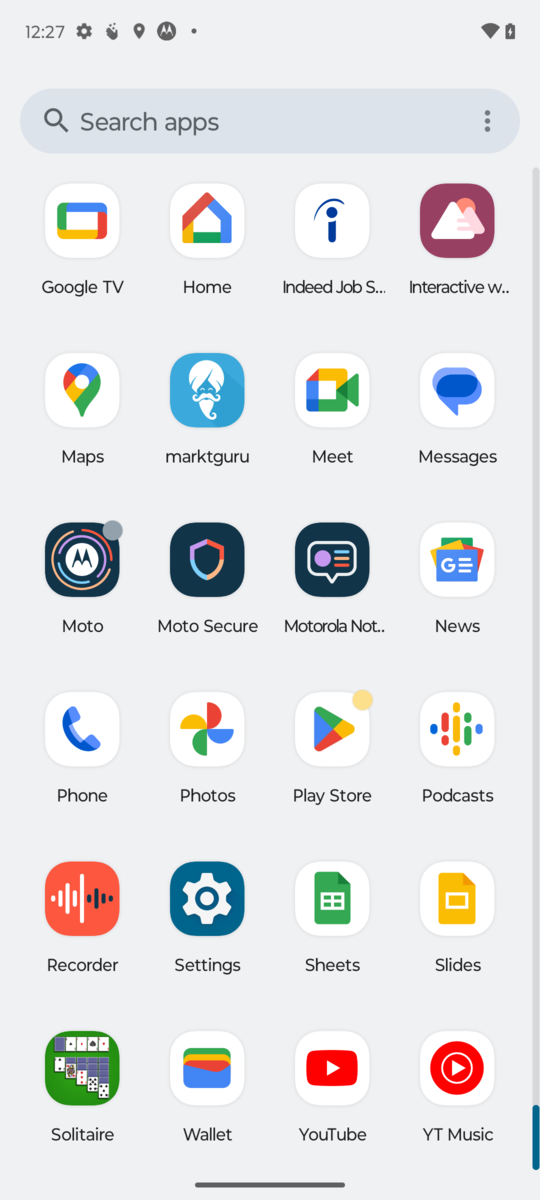This is a detailed caption for a mobile phone's home screen image:
 
The screenshot captures a mobile phone's home screen with a minimalist white wallpaper as the background. At the top, in a gray font, the current time is displayed as 12:27, followed by a series of system icons. From left to right, these include a gear icon indicating settings, a hand-shaped icon for accessibility features, a location icon signifying GPS status, the Motorola icon denoting the device brand, a Wi-Fi connectivity icon, and a battery status icon.

Beneath these icons is a darker gray search bar, with a magnifying glass icon on the left, and the text "Search apps" displayed centrally. On the far right of this search bar, there are three vertical gray dots indicating additional options.

Below the search bar, the screen is fully populated with app icons arranged in six vertical rows, each containing four apps horizontally. These apps are organized as follows:

- First row: Google TV, Google Home, Indeed Job Search, Interactive Weather.
- Second row: Maps, Mark Guru, Google Meet, Messages.
- Third row: Moto, Moto Secure, Motorola Notes, News. 

The arrangement reflects a well-organized and functional home screen, with essential and frequently used applications readily accessible.